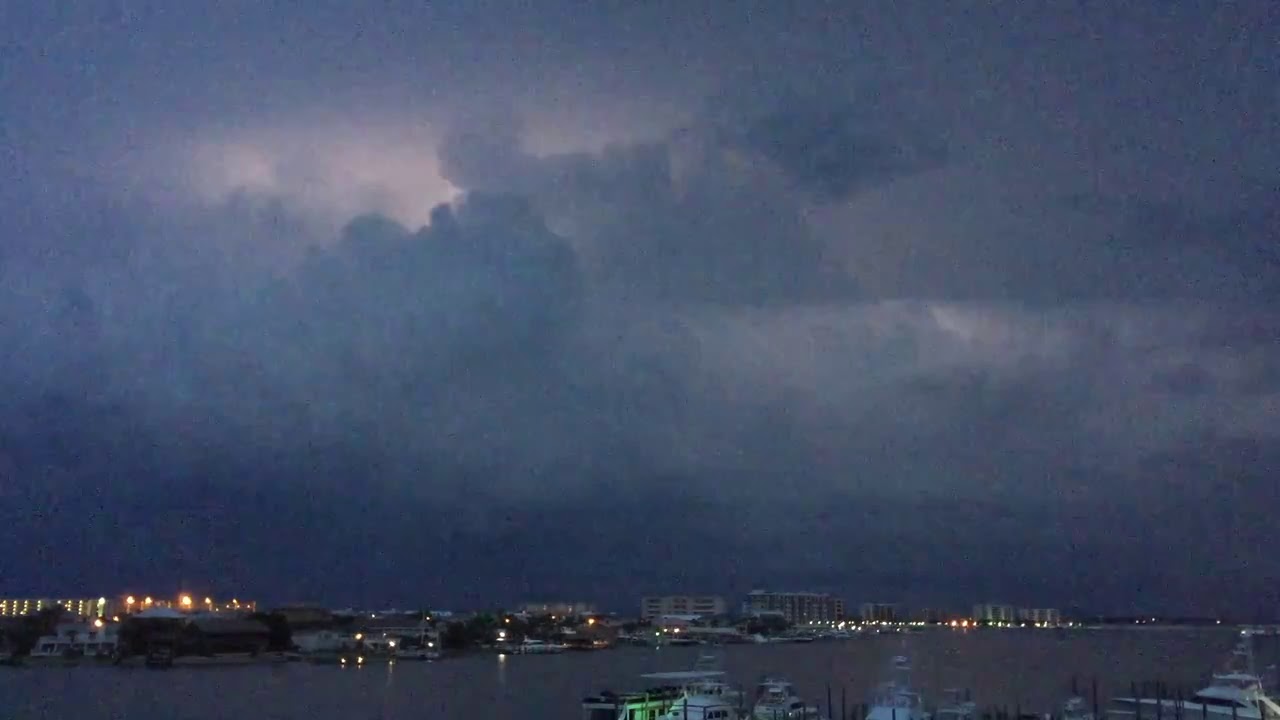The image captures an evening scene of a harbor set against an impending thunderstorm. The foreground is dotted with numerous docked boats, likely fishing boats, aligned neatly at a pier or dock. The water around the boats has a dark, purplish-blue hue, contributing to the moody atmosphere. Above, the sky is dominated by dark, turbulent clouds, with hints of lightning illuminating the upper left area, signaling the approaching storm. In the distance, a city skyline is visible on the right, populated with well-lit homes and several darker apartment buildings, suggesting a dense urban area. The sky transitions from a deep, stormy blue at the horizon to a slightly lighter shade as it stretches upward, indicating the onset of nighttime.